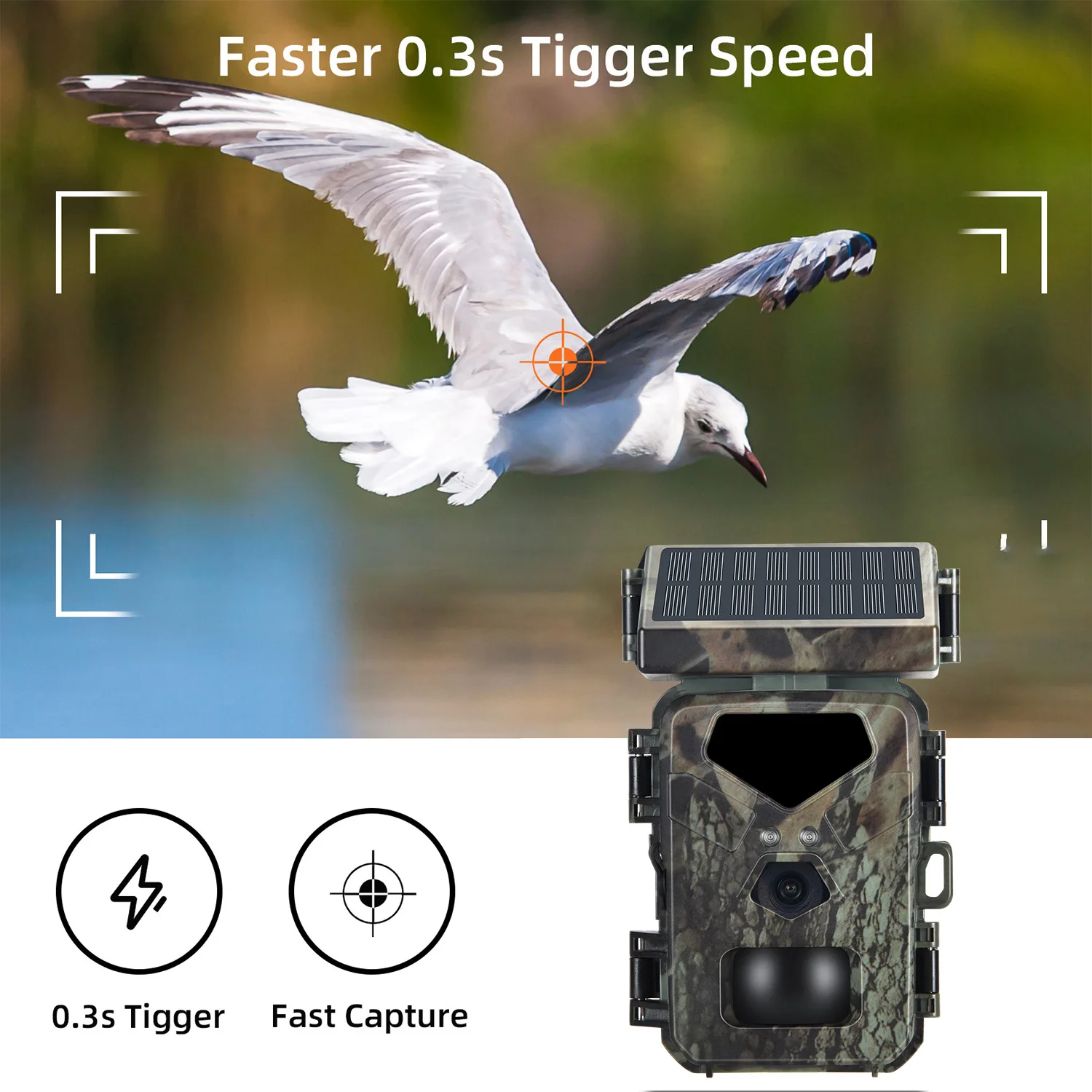The advertisement showcases a cutting-edge camera designed for fast capture. At the top, a seagull is shown in flight, with a faint green background and blurred scenery that might be a lake. The bird is glancing downward toward the center, resembling it is focusing on the advertised camera's lens. Around the bird's image, a viewfinder frame highlights the technology's precision, and above it, white text announces "Faster 0.3s Trigger Speed," emphasizing the camera's rapid response time.

Near the bottom of the image, the camera itself is prominently displayed. It's housed in a camouflage-like exterior, with a hint of a solar panel at the top for power. In the middle of the device, a rectangular foam-like section encases the lens, which is positioned centrally. To the left of the camera, circular icons are present — one depicting a lightning bolt with "0.3s Trigger" and another with a bullseye, labeled "Fast Capture." These features underscore the camera's quick detection and capturing capabilities.